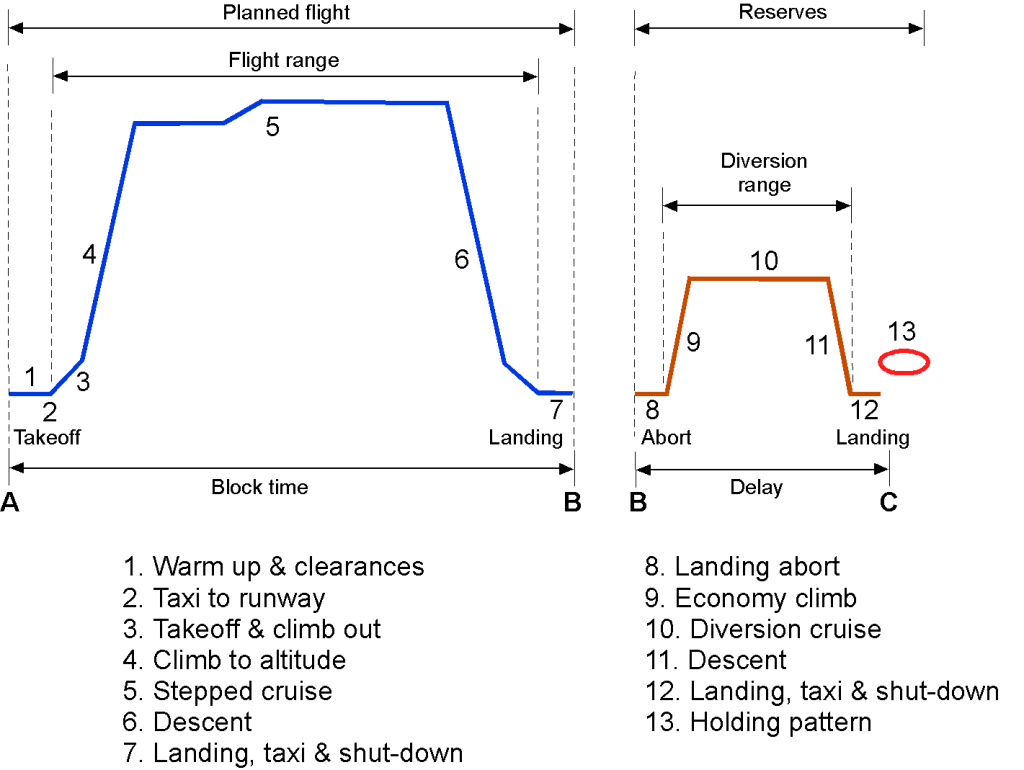This image is a detailed diagram depicting flight operations and procedures for aircraft. It comprises two main charts: a larger one on the left and a smaller one on the right. Both charts illustrate various phases of a flight from takeoff to shutdown.

The left chart is titled "Planned Flight" at the top with arrows indicating the flight path from point A (takeoff) to point B (landing). Below this, "Flight Range" is labeled, accompanied by a graph marked with a blue line and numbers from 1 to 7. These numbers represent different flight phases:
1. Warm-up and Clearances,
2. Taxi to Runway,
3. Takeoff and Climb Out,
4. Climb to Altitude,
5. Step to Cruise,
6. Descent,
7. Landing, Taxi, and Shutdown.

The smaller chart on the right is titled "Reserves" at the top, indicating a secondary flight path labeled from point B (landing) to point C (abort and landing). Below this title is "Diversion Range," and the chart is marked with numbers from 8 to 13, representing additional flight phases:
8. Landing Abort,
9. Economy Climb,
10. Diversion Cruise,
11. Descent,
12. Landing, Taxi, Shutdown,
13. Holding Pattern.

Together, these charts provide an exhaustive overview of both planned flight operations and contingency measures during diversion or delay scenarios, covering everything from initial preparation to final shutdown.